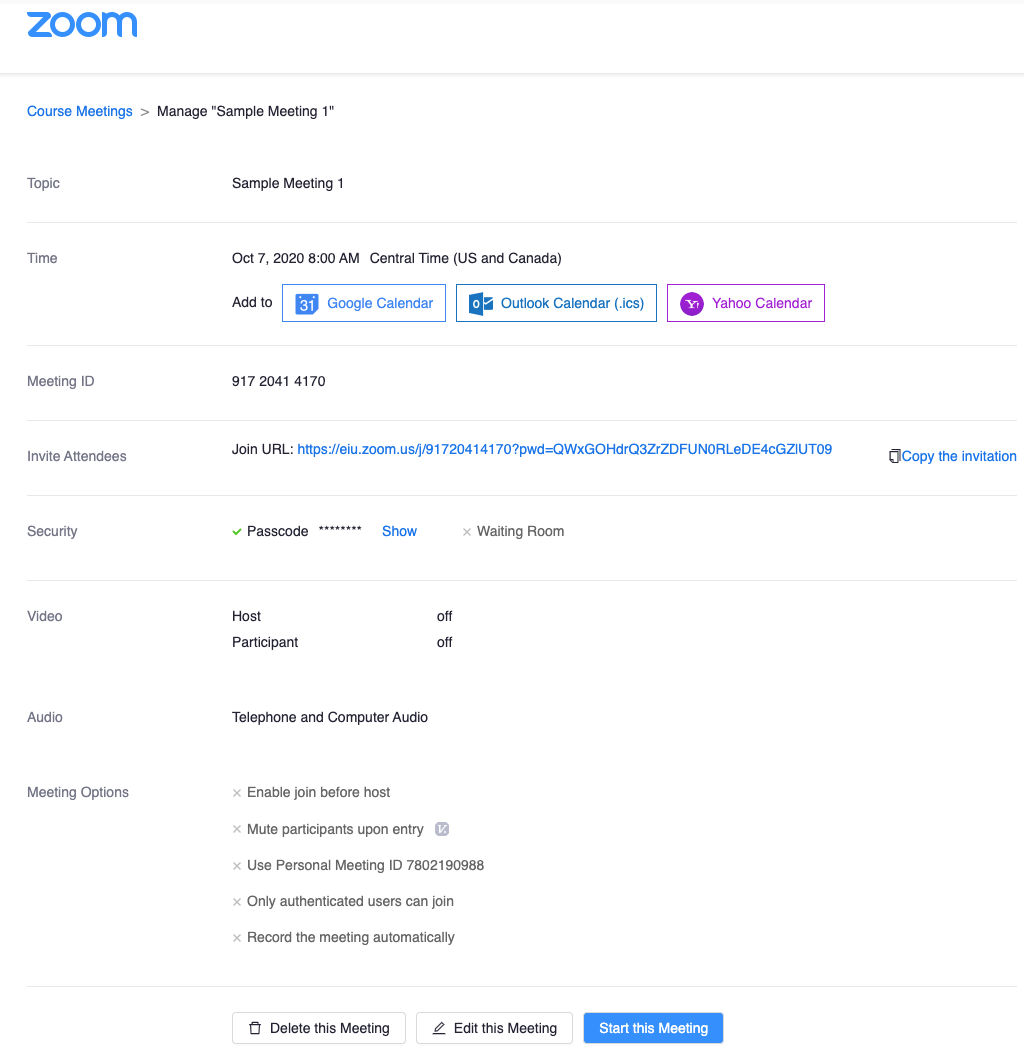The image depicts a webpage in Blueprint style, primarily focused on setting up a Zoom meeting. At the top, the word "Zoom" is prominently displayed. Directly beneath, there's a horizontal line that separates the header from the rest of the content.

Below the line, the page header reads "Course Meetings," followed by a right-pointing arrow, and the command "Manage 'Sample Meeting 1'," with the numeral one in quotes.

The next section outlines the meeting details, starting with the "Topic: Sample Meeting 1." The scheduled "Time" is specified as October 7, 2020, at 8:00 a.m. Central Time (US and Canada). Options to add this event to a Google Calendar, Outlook Calendar, or Yahoo Calendar are provided.

Further down, the "Meeting ID" is listed as 917-2041-4170. An invitation section includes the "Join URL," accompanied by a clickable link, and an option to "Copy the Invitation."

Under the "Security" heading, a green check mark implies security settings are enabled. The "Passcode" is present but obscured (indicated as starred out), with an option to "Show" the passcode in blue text. Below that, it mentions the "Waiting Room" feature with an "X," indicating it may be disabled.

The "Video" settings show that both the host and participant video options are turned off. The "Audio" settings allow for both telephone and computer audio connections.

Under "Meeting Options," several features are listed with "X" marks beside them, denoting settings turned off or unavailable:
- Enable join before host
- Mute participants upon entry
- Use Personal Meeting ID (780-2190-988)
- Only authenticated users can join
- Record the meeting automatically

Finally, action buttons at the bottom include options to "Delete this Meeting," "Edit this Meeting," and "Start this Meeting," the last of which is highlighted against a blue background.